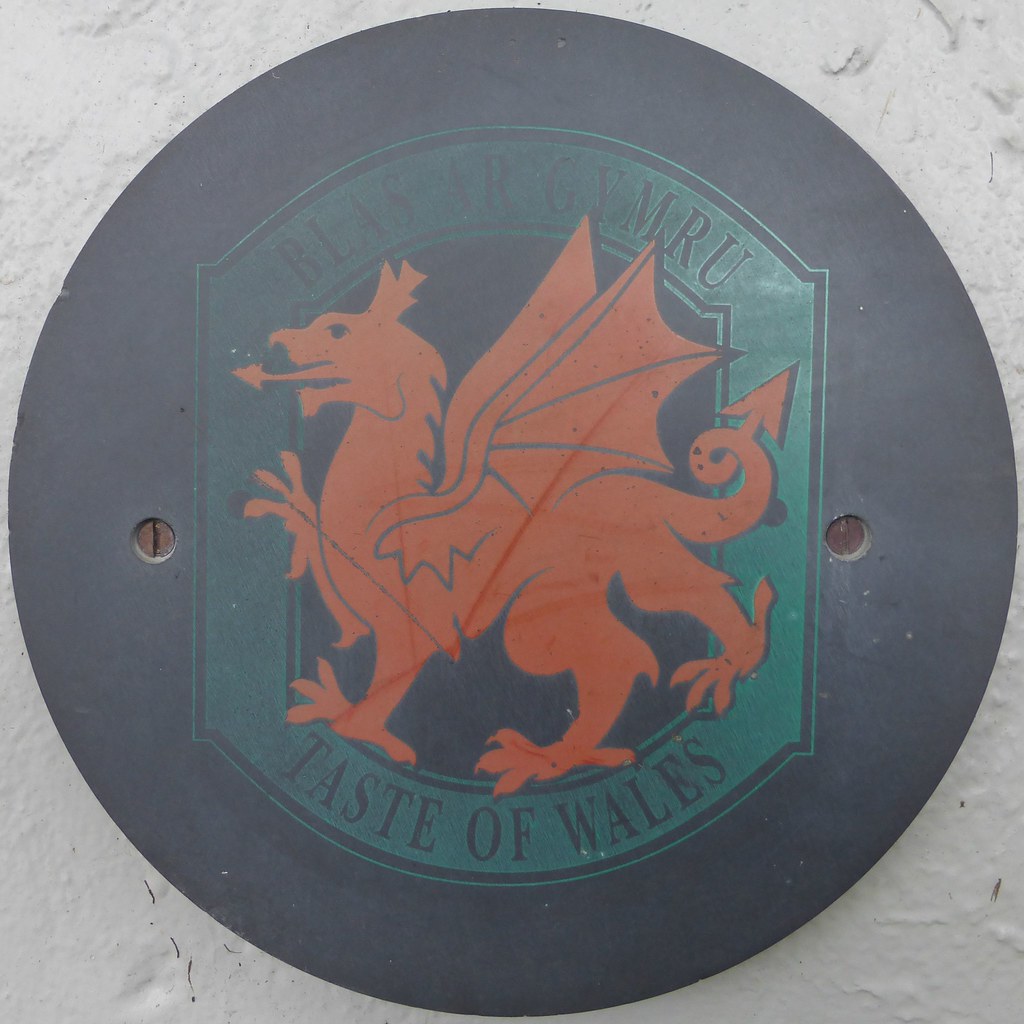The image depicts a close-up of a round, black metal plaque affixed to a white-painted stone or cement wall. The plaque features a green coat of arms emblem with an orange dragon at its center, characterized by its outstretched wings, bird-like talons, and a pointy arrow-shaped tail. The dragon, with two ears and a tongue that also comes to a point, appears to be mid-motion with one front and one rear claw lifted off the ground. Above the emblem, the text "BLAS AR GYM RU" is inscribed in black, translating to "Taste of Wales" at the bottom of the plaque. The plaque's precise detailing includes screws on either side, securing it to the wall, suggesting it might be an advertisement or a decorative marker associated with a building.